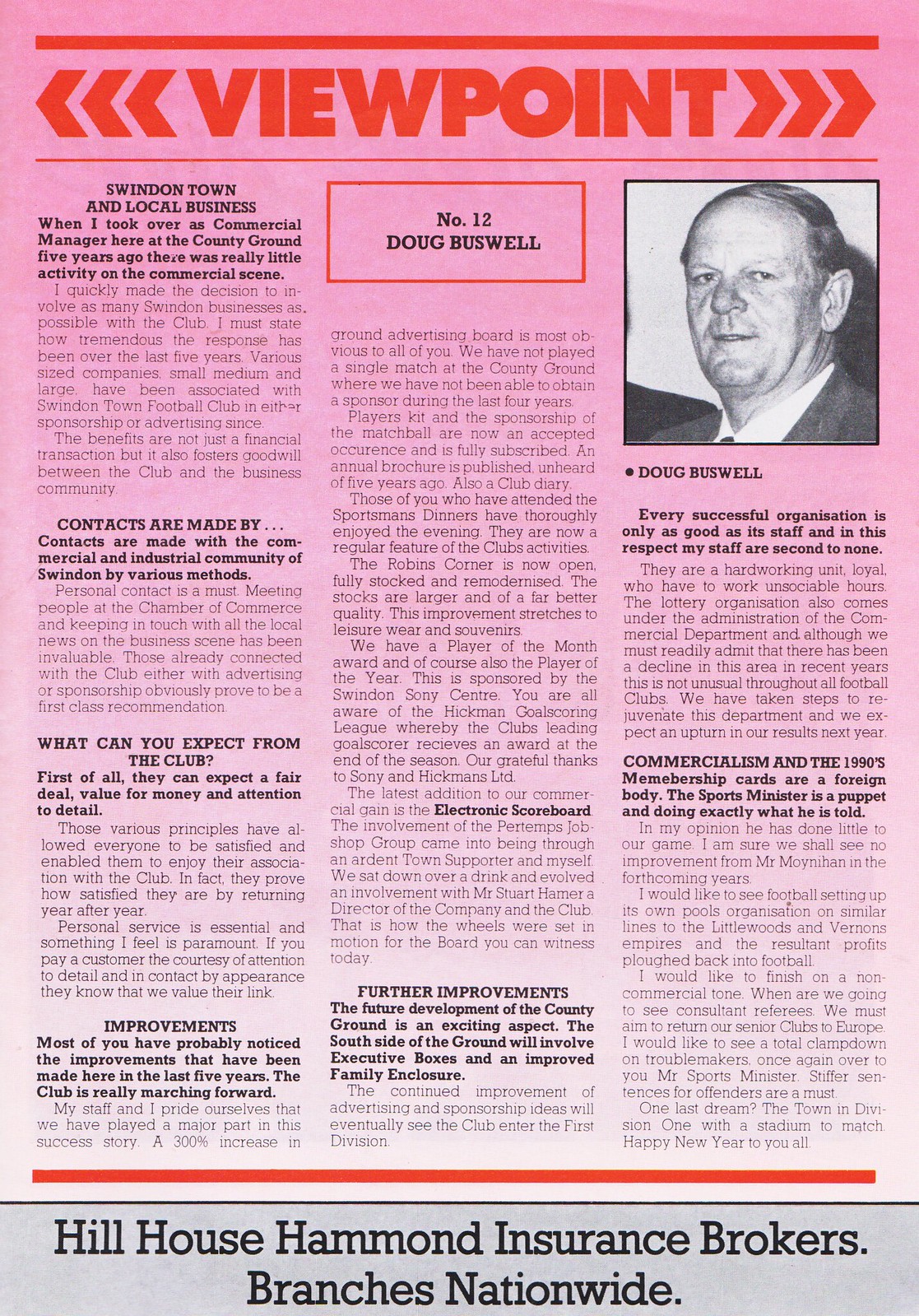The image is a detailed page from a magazine featuring a pinkish background that transitions from bright to light pink. At the top, bold red text announces "Viewpoint," with arrows extending outward on both sides. Nearby, a red box displays "Number 12, Doug Buswell." In the top right corner, there is a black-and-white photo of a man looking directly at the camera, labeled "Doug Buswell" in black text beneath it. The page is structured into three columns of black-and-white articles, with some sections highlighted in black for emphasis. At the bottom, a red stripe separates the page, transitioning into a rectangular section where bold black text states, "Hillhouse Hammond Insurance Brokers Branches Nationwide." This detailed layout and use of color suggest it is a magazine rather than a newspaper.